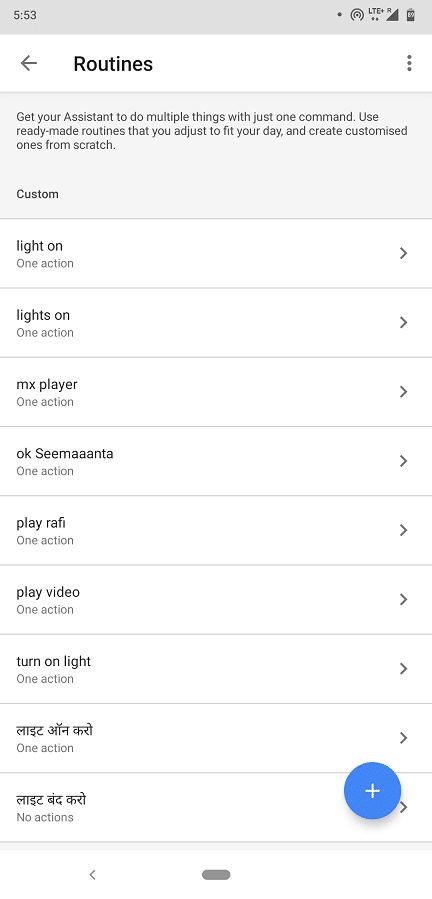This screenshot, captured from a mobile device in vertical orientation, showcases the "Routines" section within the settings menu, featuring a clean white background. At the top, there's a gray back arrow adjacent to the "Routines" title, indicating navigation to the previous menu. Below this, a gray text box provides an insightful description: "Get your assistant to do multiple things with just one command. Use ready-made routines that you adjust to fit your day and create customized ones from scratch."

The section lists predefined routines, separated by thin gray lines. These routines include:
1. "Light on" - 1 action
2. "Lights on" - 1 action
3. "MX Player" - 1 action
4. "OK Sima Santa" - 1 action
5. "Play Rafi" - 1 action
6. "Play video" - 1 action
7. "Turn on light" - 1 action
8. A routine named in an unrecognizable language - 1 action
9. Another routine in an unrecognizable language - No actions

This detailed display highlights the diverse range of available routines, each designed to perform specific tasks with a single command, emphasizing user convenience and customization.